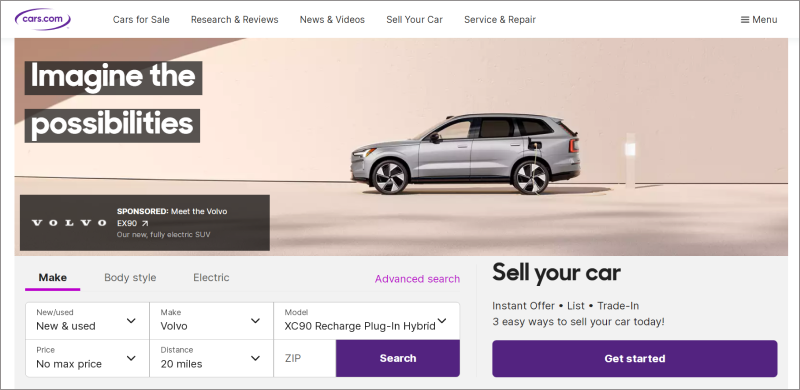This is a landscape-oriented rectangular screenshot, approximately two and a half times as long as it is wide, taken from a webpage on cars.com. The overall background of the page is white with a thin gray border around the entire image. The top section of the image features the cars.com logo in the upper left corner, which is purple and set within a white oval shape. Adjacent to this logo, there are five grey text sections: "Cars for Sale," "Research & Reviews," "News & Videos," "Sell Your Car," and "Service & Repair." All the conjunctions are represented by ampersands. In the upper right corner, there are three horizontal bars stacked vertically followed by the word "Menu," indicating a dropdown menu option.

Dominating the image is a long, landscape photo of a silver, four-door hatchback car, presumably a Volvo. The car is positioned towards the middle of the picture, facing left, with a likely electric car recharging post in the background. The backdrop of the image is a light, ambiguous color that might be a mix of grayish-brown or grayish-purple, with the car's shadow visible beneath it. The setting suggests an empty floor space with a plain wall in the background.

The top left of the car photo contains two dark gray fields with white text. The upper text reads "imagine the" and the lower text reads "possibilities." In the lower left corner, another dark gray rectangular field displays the Volvo logo in its standard font, followed by "Sponsored: Meet the Volvo X90, our new fully electric SUV."

Beneath the photograph, the lower section of the image features a light gray background. The right side prominently showcases a header labeled "Sell Your Car," accompanied by the caption "instant offer · list · trade-in – Three easy ways to sell your car today." Beneath this, a purple rectangular button with white text that reads "Get Started" is displayed.

Occupying roughly 60% of the lower section on the left are three searchable categories: "Make," "Body Style," and "Electric." The "Make" category is currently selected and highlighted in dark gray bold text with a purple underline. Advanced search options are marked in lavender in the upper right. Below these categories, three columns and two rows of selection fields are presented, each with a downward-facing arrow for dropdown selections. The fields display options such as "New & Used," "No Max Price,” “Volvo,” “20 miles,” “XC90 Recharge Plug-In Hybrid,” and an empty "ZIP" field for entering a postal code. To the right of these fields, a purple button with white text labeled "Search" is situated.

This detailed description captures the overall layout and key elements of the cars.com page depicted in the screenshot.